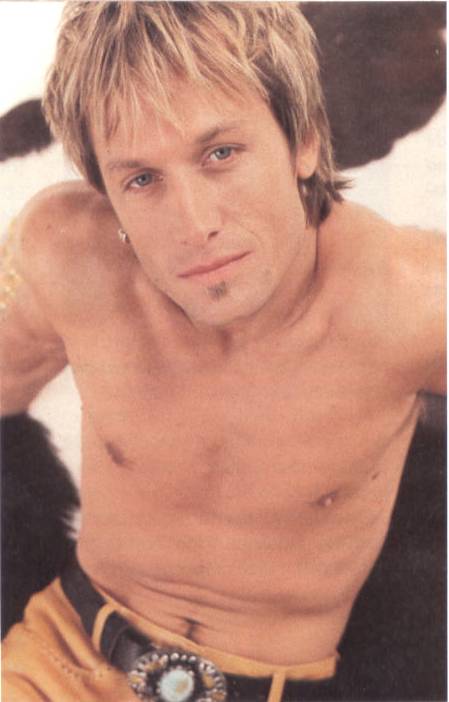The photo features a shirtless white male with sandy, dark blonde hair styled in a long, shaggy, and spiky manner. He has a diamond stud earring in his right ear. The man wears yellowish-gold jeans paired with a black leather belt, which sports a distinctive silver buckle adorned with a white opal-shaped centerpiece surrounded by a black ring. Centered in the image, he sits on a fuzzy, black-and-white surface that could be a bear skin rug, a cow print rug, or perhaps even an asphalt road, suggesting an outdoor setting, possibly in the middle of the day. The background colors of the image include black, gray, tan, and light brown. Additionally, he has a small square patch of hair directly below his bottom lip.